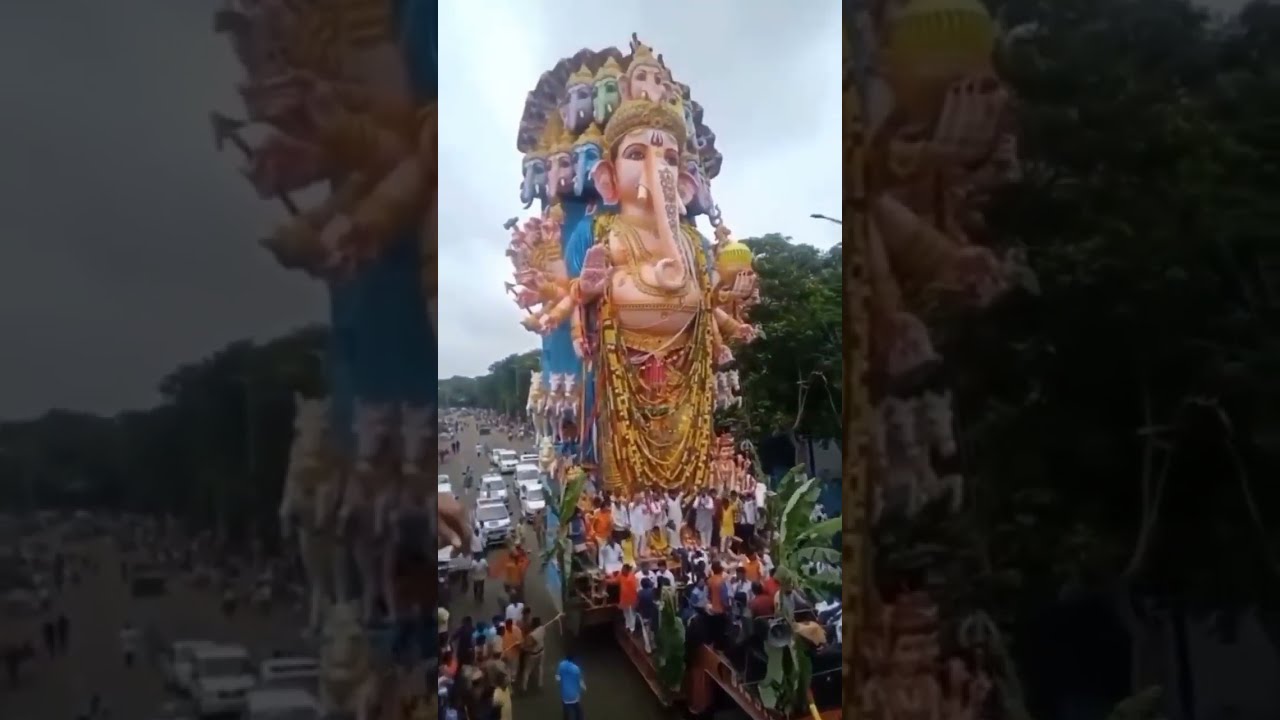The image depicts a grand and elaborate float at a parade, showcased in a vertical, cell phone-style photograph with zoomed-in, faded replicas on either side. At the center of the float stands a towering and imposing statue of a Hindu deity, specifically Lord Ganesha. This statue features a human-like face with an elephant trunk, large ears, a sizable belly, and multiple hands, each holding different objects or ornaments. It is adorned with a gold or gold-and-orange cloth that drapes down and is also wearing a distinctive knitted-style hat.

The deity's forehead is marked by a three-pronged fork symbol. Surrounding the feet of this immense statue are dozens of devotees and participants, some carrying the structure, reflecting the fervor of the Ganesh Chaturthi celebration in India. The street is filled with people and bordered by a row of green-foliaged trees. The sky above is overcast with grey clouds, contributing to a subdued atmosphere. Vehicles and additional people can be seen in the background, all contributing to the vibrant yet chaotic scene of the outdoor procession.